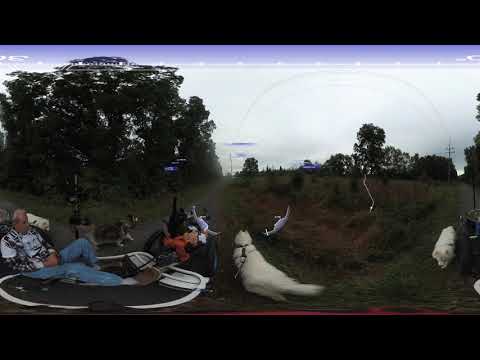The image captures a skewed, panoramic outdoor scene with noticeable graininess and distorted proportions due to the 360-degree angle. Central to the image are at least three individuals, including an older man seated on the ground in jeans and a black-and-white textured long-sleeve shirt. His right leg is outstretched while his left leg is bent, and his hands rest in his lap. Surrounding him are a few trees and a grassy area, indicating a park-like setting. There are at least four dogs present: two white and two black or gray. One white fluffy dog, wearing a collar and leash, is positioned towards the bottom center of the image, facing away. Another dog is to the right of the man, and in the background, one dog is rolling on its back while another walks toward the camera. Adding to the complexity of the image, the top features some white text, though its content is unreadable. Black bars frame the top and bottom of the image, enhancing the sense of a panoramic view with circular warps on the left and right sides.